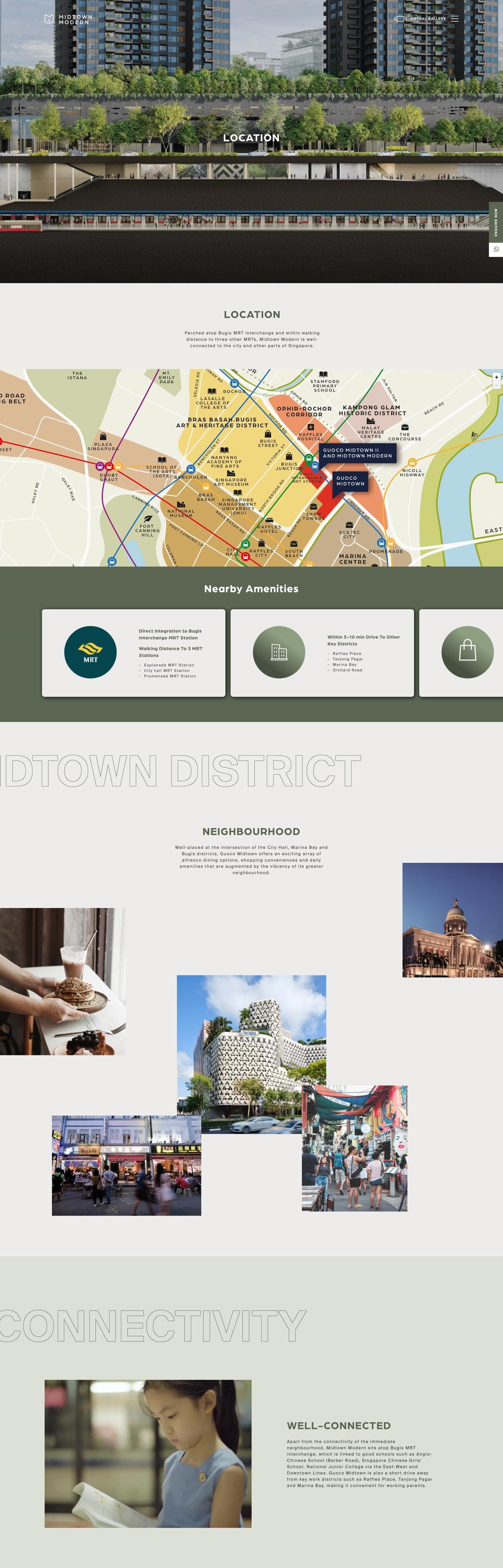This image appears to be a detailed screenshot of a website layout. At the top, an image banner displays skyscrapers under a grey sky with trees in the foreground. The banner also features a slim black strip in the middle, containing some white text that is difficult to read due to its small size.

Beneath the banner, the background transitions to white and showcases a map. The map includes water bodies to the right and left, and various colored land blocks in the center, including shades of brown, greyish brown, yellow, and red. Some black boxes are scattered across these colored blocks, possibly indicating specific points of interest.

Further down, there's a dark green horizontal band featuring white rectangles with black text. Within this band, on the far right, there are two green ovals with white text inside them. To the far left of this band, there is a darker green oval containing a yellow and white logo.

The lower section of the image is divided into additional panels. The first is a white panel with some black text in the middle, which is surrounded by five photos. These images include:
1. A person's hands on a table holding a drink.
2. A skyscraper in the center.
3. Another building against a blue sky on the right.
4. A street scene beneath the previous building photo on the right.
5. What appears to be a vehicle on the left, though the details are indistinct.

At the very bottom of the screenshot, a green background contains what looks like a watermark or text that may read "Code Collectivity" or something similar to that. Overlaying the white background portion of the image is similar text, partially legible as "digital." 

In the lower right-hand corner, there is a picture of a young girl with light brown skin reading a book. She is wearing a sleeveless blue top or dress and is accompanied by some black text to her right.